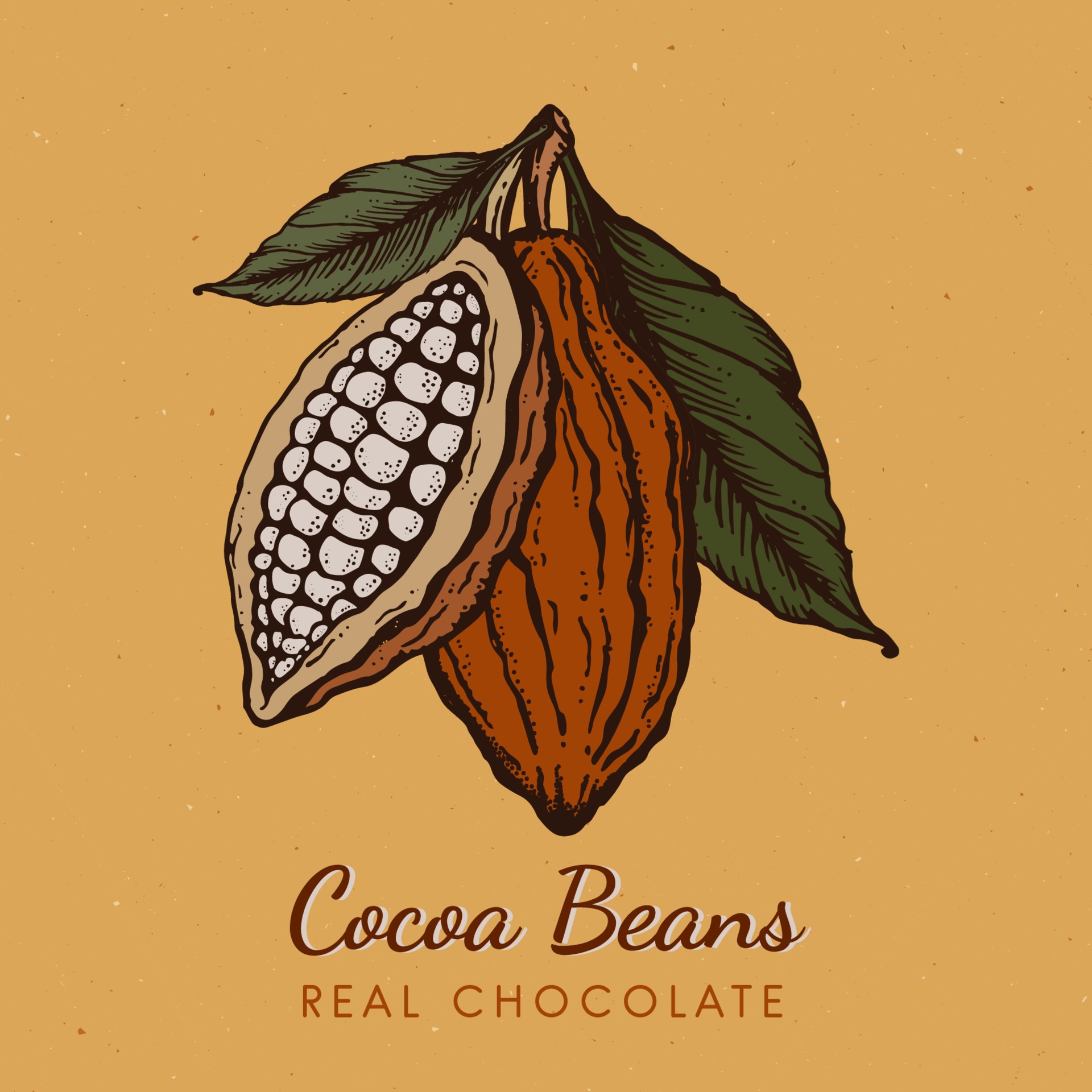This image is a detailed color illustration of a cocoa plant, rendered with a slightly grainy, light brown, and orangey background. At the center-top of the square format image, two cocoa pods are attached to a single branch, accompanied by two dark green leaves—one leaf extends toward the bottom right and the other toward the top left. The pods consist of one whole pod with a brick red-brown exterior marked by black lines, and a partially open pod at an angle revealing its interior. Inside the sliced pod, rows of white, teeth-shaped seeds are visible against a dark background, lined with cream-colored shell edges. Beneath the illustration, the text reads "COCOA BEANS" in dark brown cursive script, and "REAL CHOCOLATE" in smaller, lighter brown block letters, both with a white border for clarity.